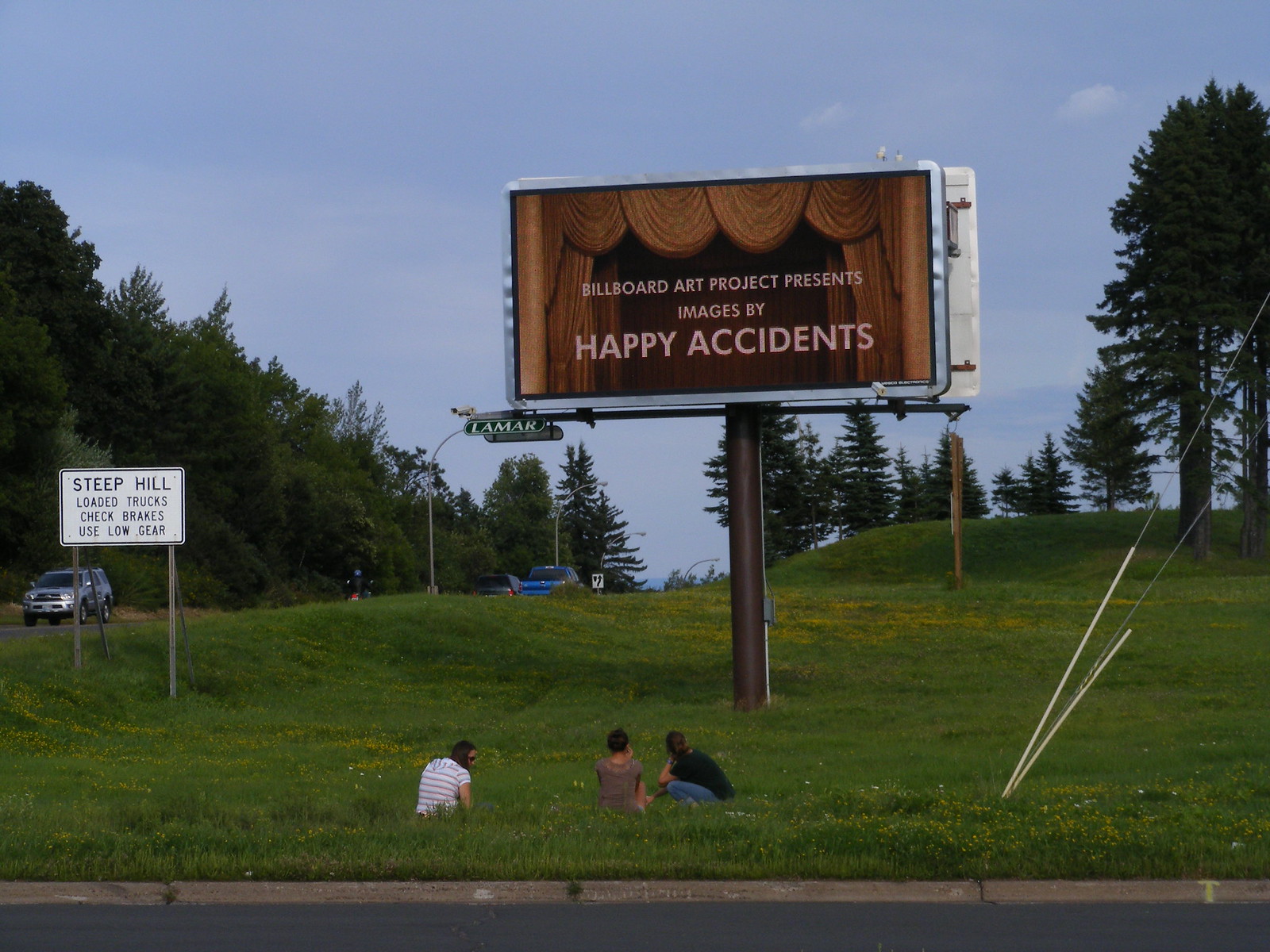A vibrant color photograph captures a group of three people sitting on a grassy hill at an intersection, gazing up at a prominent billboard. The billboard, supported by a long brown pole, features a golden-brown stage curtain with the text, "Billboard Art Project presents images by happy accidents," centered on it. In the background, lush green hills rise to the right, leading up to more trees, while additional trees and a few streaky white clouds are visible against the blue sky. To the left of the billboard, a traffic sign reads, "Steep Hill, Loaded Trucks, Check Brakes, Use Low Gear." The scene is lively, with cars driving along the adjacent street and a visible curb marking the edge of the road. A cable with white protective covering runs into the ground on the right side, adding to the detailed snapshot of this idyllic outdoor setting.